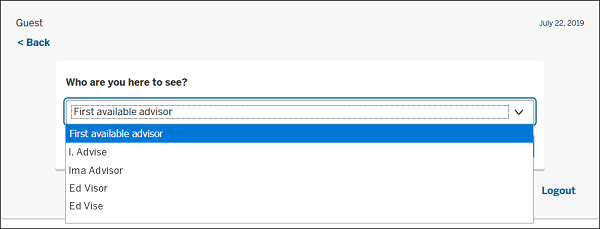The digital image depicts a user interface screen. At the top left corner, a drop-down button labeled "Guest" is visible. Right next to it, there's a "Back" button featuring a blue arrow. In the top right corner, the date "July 22, 2019" is displayed.

Beneath this, a prompt in bold black font asks, "Who are you here to see?" Below this question, there are several options visible:

1. "First available advisor" - This option is highlighted in blue and appears twice on the screen.
2. "1. Advise" - This appears below the first option.
3. "I am an advisor" - Listed as another selection.
4. "ED advisor" - This is another available option.
5. "ED advise" - Listed as the final option.

In the bottom right corner of the screen, there is a "Log out" button presented in dark blue font.